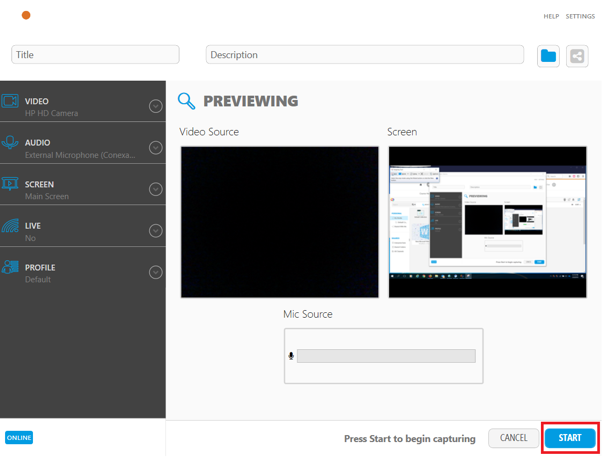In this detailed image, the left side features a navigation bar set against a black background. At the top, there is a text label that reads "Video HP HD Camera," accompanied by a blue video camera icon on its left. Directly beneath it, the item "Audio" is listed with a blue microphone icon next to it. Further down, the options "Screen," "Main Screen," and "Live" appear sequentially, with "Live" having the word "No" under it, accompanied by a pull-down arrow on its right. Following this, the caption "Profile" appears with an icon of a person from the waist up and another pull-down arrow to the right. Below "Profile," the text reads "Default." Near the bottom of the navigation section, a blue button labeled "Online" is prominently displayed.

On the lower right corner of the screen, in black text, there is an instruction that reads "Press Start to begin capturing." To the right of this instruction are two action buttons: the first one is white and labeled "Cancel," while the second is a blue button with white text that says "Start," outlined with a red square.